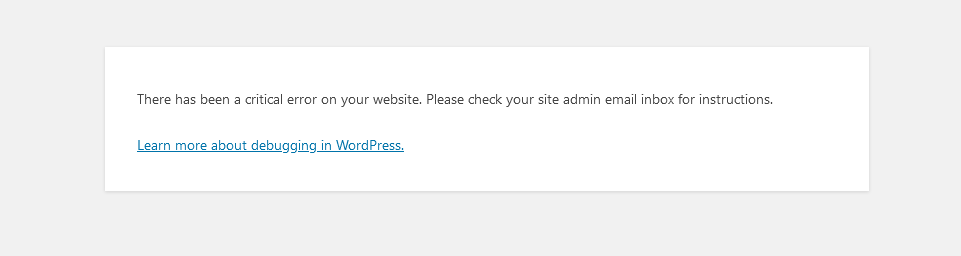The image features a simple, clean design with a light gray background. Centrally positioned within the gray area is a white, rectangular box. This white box occupies the middle portion of the image, providing a focal point. Inside the box, the content is arranged with ample spacing, giving it a neat and organized appearance. 

The text within the box includes two sentences and a hyperlink below them. The sentences read: "There has been a critical error on your website. Please check your site admin email inbox for instructions." Beneath these sentences, there is a link that says, "Learn more about debugging in WordPress." The overall layout is straightforward and functional, clearly conveying the message about the website error and providing a call-to-action for further assistance.